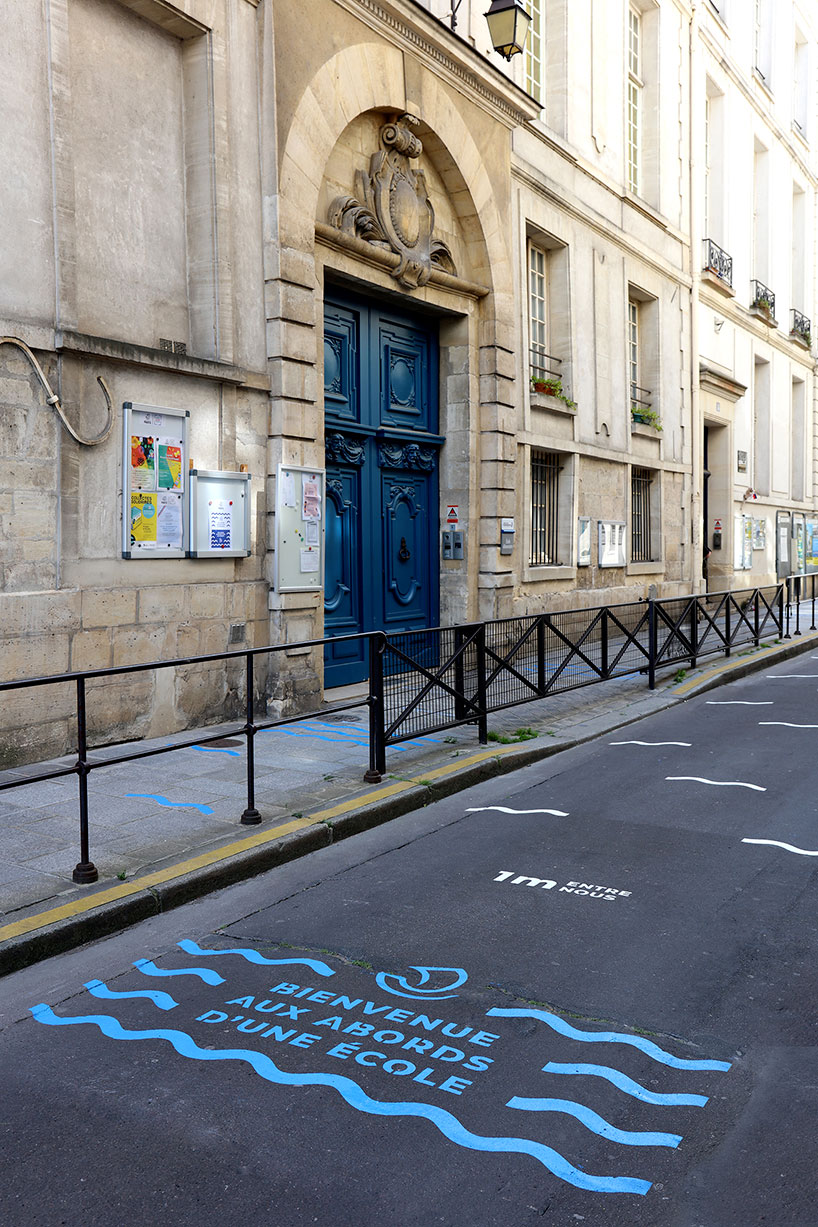This photograph captures a French street scene, with a dark gray asphalt road running diagonally from the bottom left to the middle right. Near the lower left corner, wavy blue lines decorate the pavement alongside white text reading "1M." Prominently displayed in the middle of the road are the words "Bienvenue aux Abords d'Une Ecole," accompanied by additional blue wave decorations. To the left of the road, a light gray sidewalk also features the same blue wavy lines. A black metal railing runs along the right of the walkway, likely serving as a safety barrier.

To the left of the image stands a large, ornate stone building with an architectural archway entrance. The doorway is richly ornamented and features a striking matte black double door. Above the entrance and along the façade, numerous windows are visible, including another entrance with windows above it. The building's stone exterior combines elements of gray stone, plaster, and beige, enhancing its grand appearance.